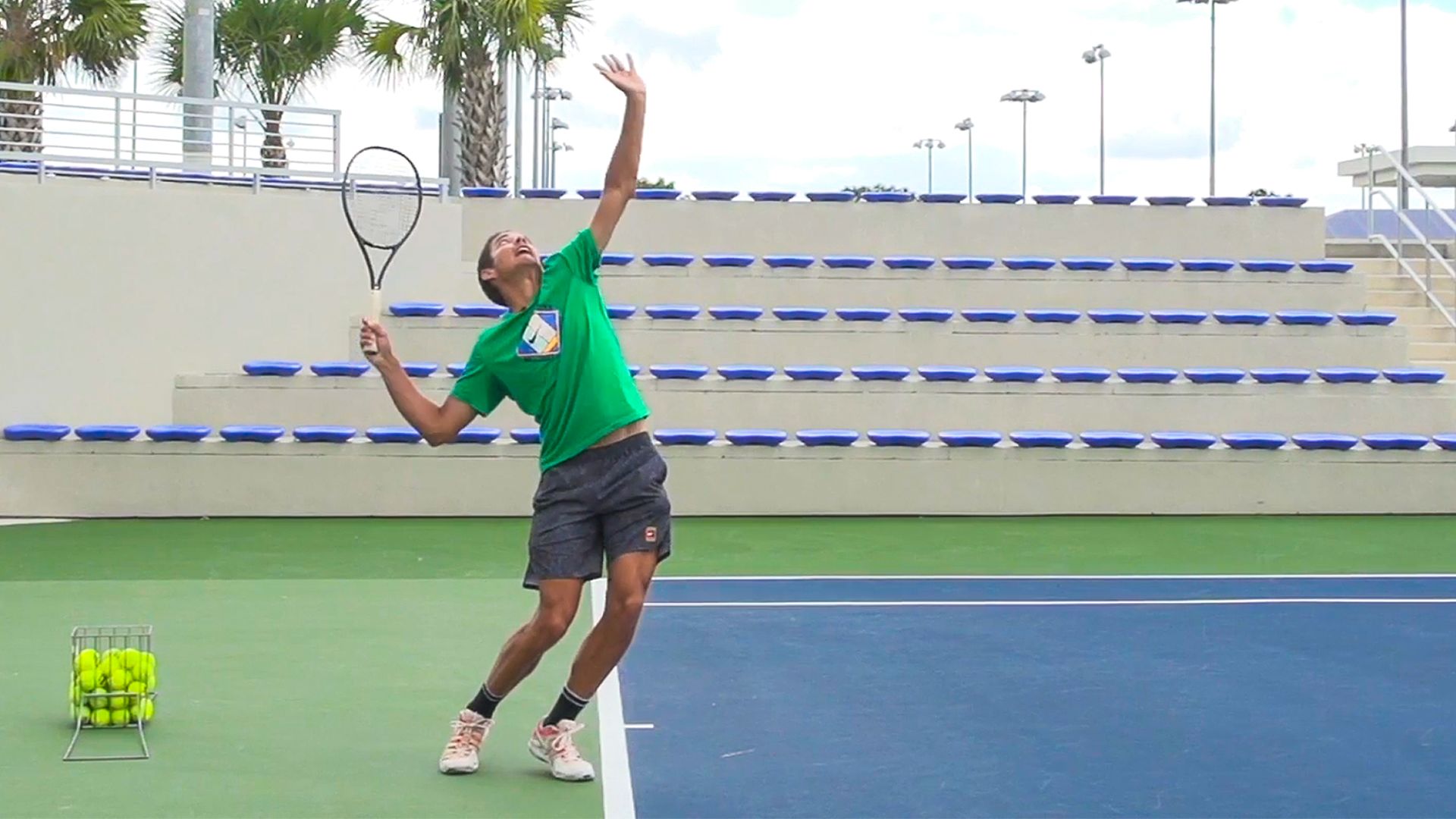On a cloudy day at an outdoor tennis court, a man is captured mid-serve, poised to hit a ball he has just tossed into the air. The blue tennis court is bordered by green turf, and white lines mark the playing area. The player, slightly bent to the left with knees flexed, is dressed in a green short-sleeved shirt, dark gray shorts, black socks, and white sneakers. His left arm is fully extended upward, palm open, while his right hand grips the racket, elbow bent in preparation for the strike. Behind him, a wire container filled with tennis balls sits on the ground. In the background, blue seats are arranged in about five rows on concrete bleachers, which are currently empty. Palm trees and streetlights are visible in the distance, beneath a mostly white, cloud-covered sky, with occasional patches of blue peeking through.